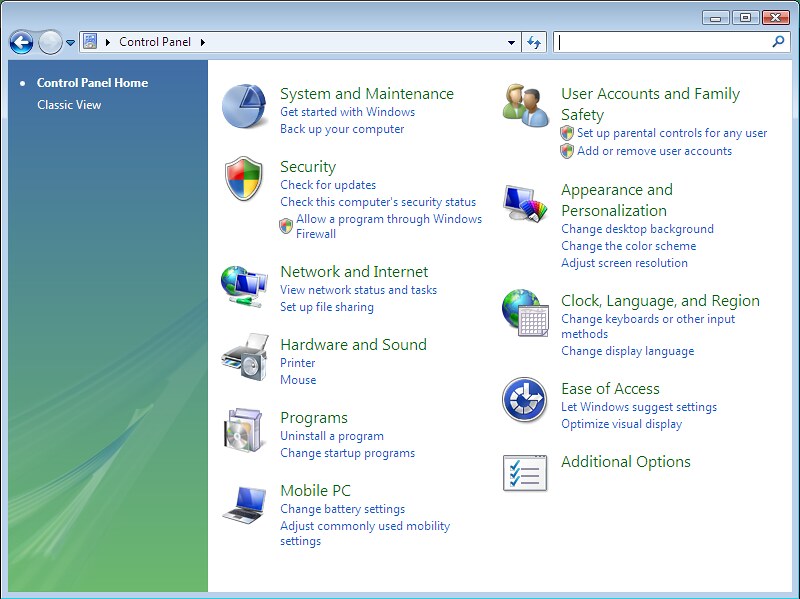The image is a color screenshot of a Windows PC Control Panel displayed on a monitor with a light blue border. At the top is a banner containing an address bar that says "Control Panel" on the left, alongside back navigation and a solid gray icon. In the upper right corner, it features the standard window control icons: minimize, restore/maximize, and close (red X).

Below the top border, the interface is divided into two main columns. On the left, there is a vertical, greenish-blue panel labeled "Control Panel Home" in white, followed by "Classic View." This panel contrasts against the general white background of the control panel.

The control panel's interface displays various sections with descriptive icons to their left. In the left column, the sections are listed as follows:
- **System and Maintenance:** Options like ‘Get started with Windows’ and ‘Backup your computer’
- **Security:** Tasks including 'Check for updates' and 'Allow a program through Windows Firewall'
- **Network and Internet:** Options such as 'View network status and tasks' and 'Set up file sharing'
- **Hardware and Sound:** Selections for 'Printer', 'Mouse', etc.
- **Programs:** Choices like 'Uninstall a program' and 'Change startup programs'
- **Mobile PC:** Settings for 'Change battery settings' and 'Adjust commonly used mobility settings'

The right column continues with:
- **User Accounts and Family Safety:** Features like 'Set up parental controls for any user' and 'Add or remove user accounts'
- **Appearance and Personalization:** Options to 'Change desktop background', 'Change the color scheme', and 'Adjust screen resolution'
- **Clock, Language, and Region:** Settings for 'Change keyboards or other input methods' and 'Change display languages'
- **Ease of Access:** Features such as 'Let Windows suggest settings' and 'Optimize visual display'
- **Additional Options**

Each section in both columns is associated with specific icons to its left, enhancing visual guidance through the options available in the standard Windows Control Panel.